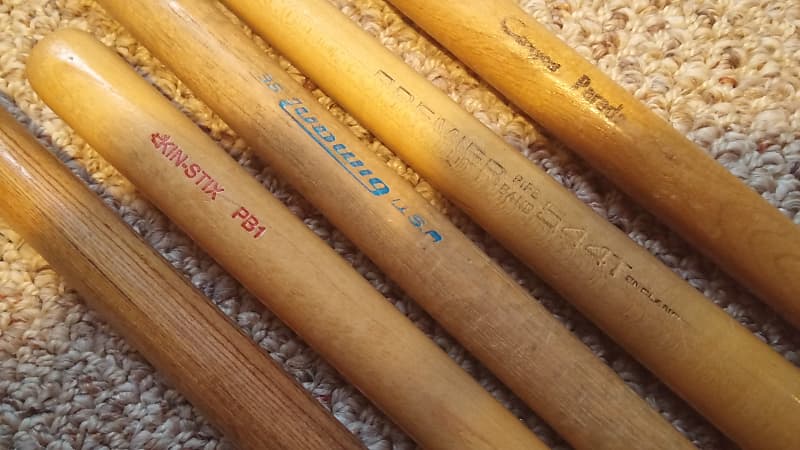This photograph showcases a collection of five vintage wooden baseball bats, arranged diagonally from the bottom right to the top left against a low-pile beige carpet with visible weave patterns. The bats exhibit notable wear, including dents, stains, and faded lettering, indicating they were likely made many years ago, prior to the advent of aluminum bats. Each bat varies in length and features distinct engravings: 

1. The top bat has a black engraving reading "CANYOTE PARADE", though the first word's lettering is faint.
2. The second bat below it has partially legible engravings, displaying the numbers "44T".
3. The middle bat bears faint blue text, with the word "USA" discernible.
4. The fourth bat features red text stating "KIN-STIX PB1" and its round tip is visible in the photograph.
5. The bottom bat is plain with no visible lettering, showcasing only the natural grain of the wood.

Soft shadows fall to the right of the bats, adding depth to the image and highlighting their aged and well-used condition.